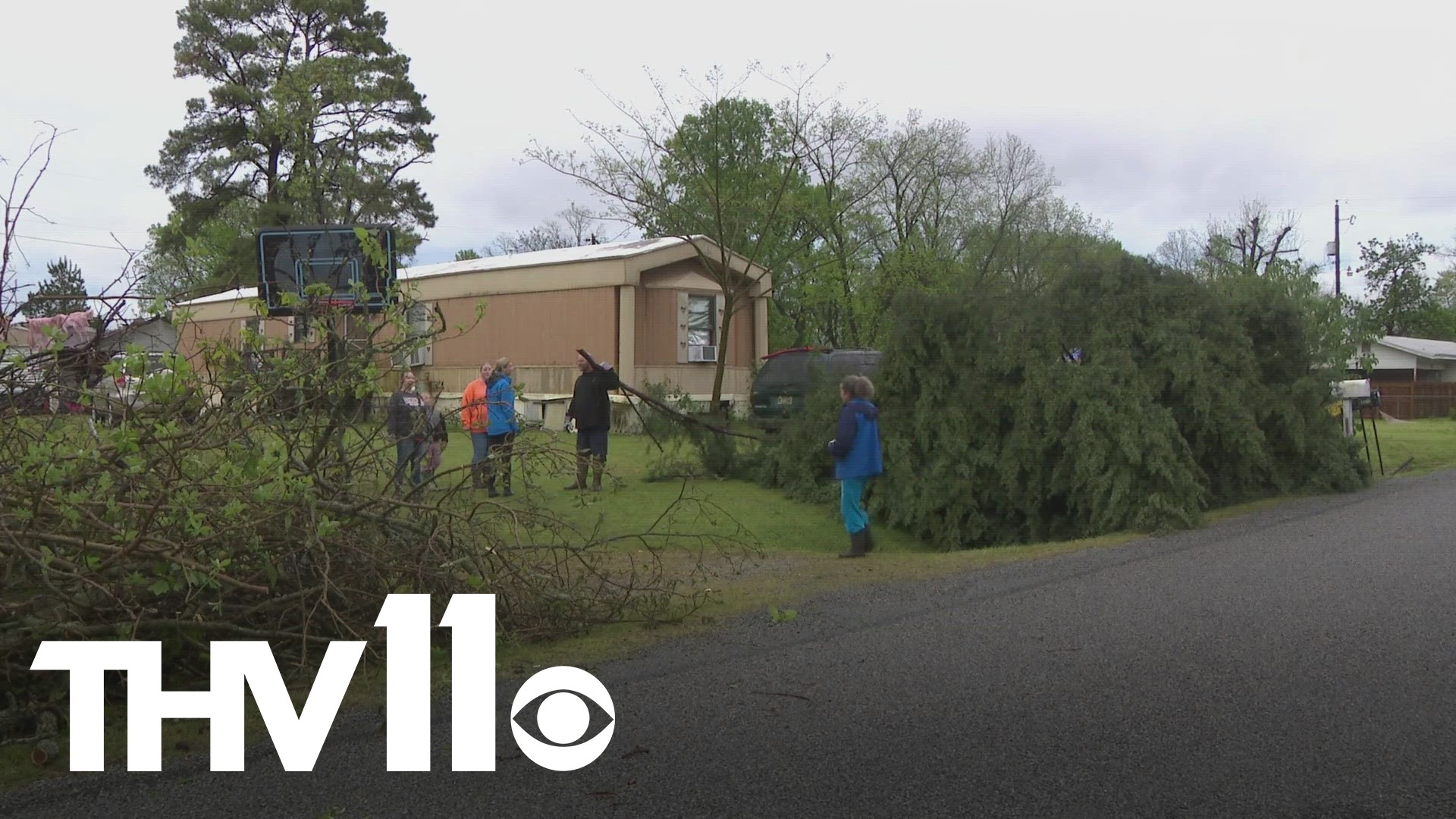The image, appearing to be a video still from local CBS affiliate THV-11, shows the aftermath of a storm with several people inspecting the damage. In the lower left corner, the image is labeled with "THV-11" and a CBS eye logo. The foreground features a dark gray paved road, while a light brown trailer with windows, including an obscured one, and an air conditioning unit, stands behind a tangle of broken tree branches. The image captures six individuals actively assessing the scene; one person, in a black shirt and blue pants, holds up a large branch while others, dressed variously in blue jackets, long curly hair in a ponytail, and colorful attire, assist or observe. Beside the trailer, there's a basketball hoop and several other fallen trees. A white mailbox, a black SUV, and a wood fence are visible in the vicinity. Overhead, the sky appears cloudy and white.